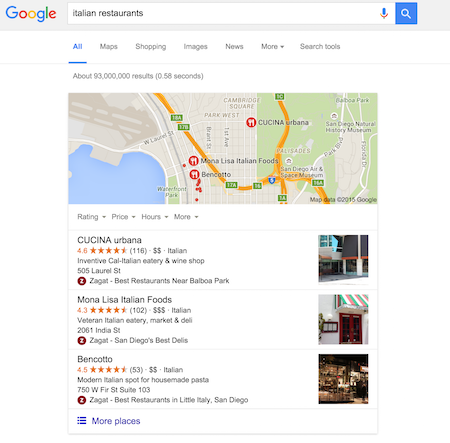The image showcases the Google search interface for "Italian restaurants." At the top, in a light gray banner, "Google" is displayed prominently. Below the banner, there is a long white search bar with the text "Italian restaurants" aligned to the left. Adjacent to this, there is a colorful microphone icon, and further to the right is a blue square containing a magnifying glass icon, signifying the search function.

Directly underneath the search bar, a navigation menu is visible. It starts with the options: "All," "Maps," "Shopping," "Images," "News," followed by a "More" dropdown arrow. "Search tools" is also listed. In this menu, "All" is highlighted in blue, indicating the active search category.

Below this navigation, a section provides results information, though some numbers are not clearly legible. A map occupies the next portion of the interface, marked with circles containing fork and knife icons that denote restaurant locations. The map also features a representation of a body of water and yellow lines indicating highways.

Under the map, there are three displayed rows, each featuring media images of different establishments on the right side, accompanied by titles on the left.

1. The first row highlights "Cucina Urbana," along with its rating and additional information.
2. The second row shows "Mona Lisa Italian Foods," boasting a 4.3-star rating.
3. The third row features "Vencata" or "Cotija" with a 4.5-star rating.

Each row contains further details about the respective Italian restaurant establishments.